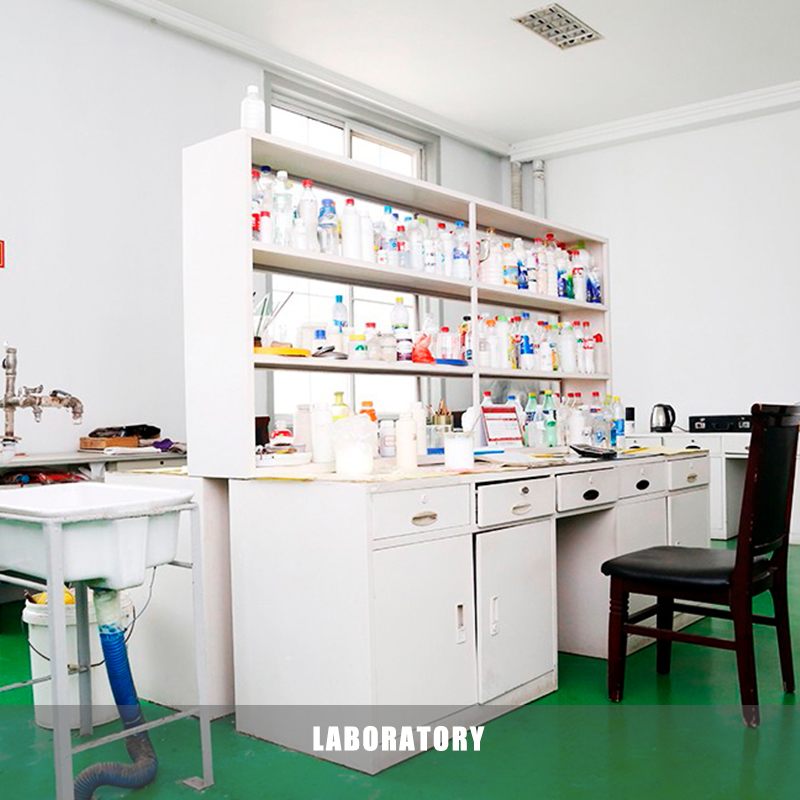The image depicts a brightly lit, well-organized laboratory room with white walls and green flooring. Prominently displayed at the bottom center of the image is the word "LABORATORY" in white, capitalized text on a thin, very pale black bar. To the left side of the image, there is a portable sink with a blue tube connected to it, and a white trash bin situated below. Adjacent to the sink, a white basket with a similar tube setup is visible, likely designed for draining liquids. In the foreground, a large white desk features five pull-out drawers with cabinet doors below them and a variety of chemistry bottles, a calculator, papers, and a chart on its surface. Above the desk, a shelving unit with six shelves is filled with bottles of different sizes and cap colors including red, blue, green, and yellow. A brown chair, possibly with a leather seat, is positioned in front of the desk. To the right edge of the image, another table holds a coffee mug and a black briefcase. The laboratory is well-lit by natural light, adding to the clarity and brightness of the scene.